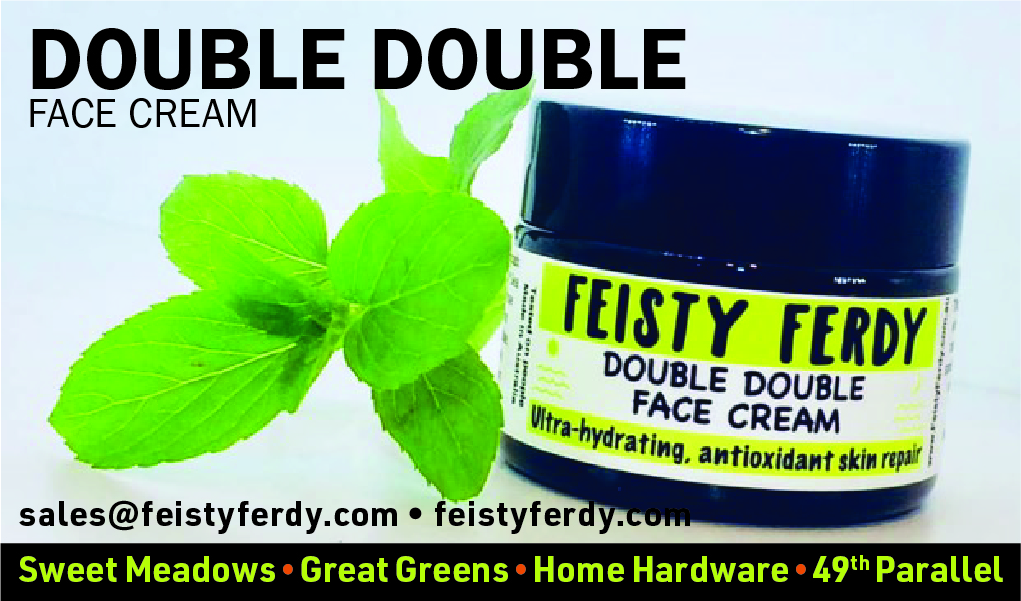This is an advertisement for Double-Double Face Cream by Feisty Ferdy. The ad features a muted bluish-gray background. Prominently displayed on the top left is the product's name in dark lettering: Double-Double Face Cream. On the bottom right, there is a navy blue jar with a dark top, adorned with a white label. The label sports yellow banners, featuring the text: "Feisty Ferdy Double Face Cream Ultra-Hydrating Antioxidant Skin Repair." Complementing the jar, to its left, is a vivid green frond with five leaves. The URL "sales@FeistyFerdy.com" is also visible. At the very bottom, a black banner lists various purchase points in yellow lettering: Sweet Meadows, Green Greens, Home Hardware, and 49th Parallel.